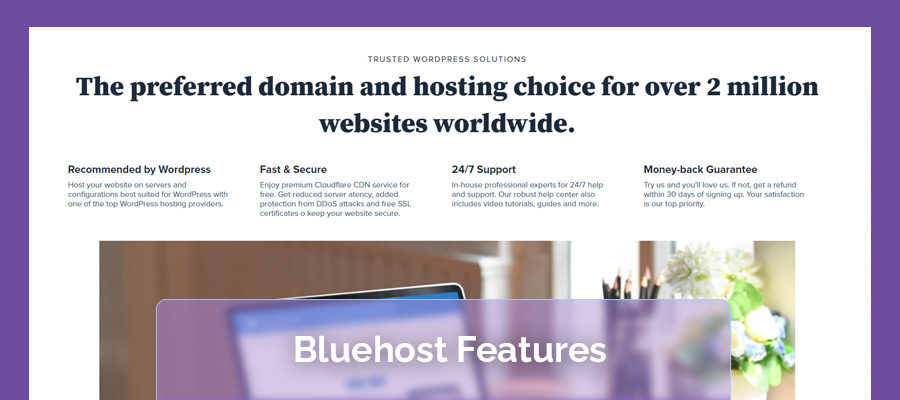**Image Caption:**

A webpage featuring a sleek and modern design, prominently displaying the header "Trusted WordPress Solutions" at the top. Encircling the content on the right, left, and top sides is a vibrant purple border, contrasting with the unbordered bottom edge. The main headline reads, "The preferred domain and hosting choice for over 2 million websites worldwide," exuding a sense of reliability and trust.

On the left side of the page, a smaller font highlights, "Recommended by WordPress. Test your website on servers and configurations suited for WordPress with one of the top WordPress hosting providers." Adjacent to it, another section boasts, "Fast and secure, enjoy premium CloudFlare CDN service for free, get reduced server latency, added protection from DDoS attacks, and free SSL certificates to keep your website secure."

Further down, a segment titled "24-7 support" assures users of round-the-clock assistance with in-house professional experts. It also mentions a robust help center that includes video tutorials, guides, and more. Finally, the "Money back guarantee" emphasizes customer satisfaction with a promise of a refund within 30 days if not satisfied.

At the bottom of the page, a somewhat transparent purple rectangle displays the text "Blue host features." The background of the webpage showcases a warm, inviting scene: a desk with a laptop, a cup containing pencils, a flower in a vase, all set against a rich brown backdrop, creating a harmonious balance of professional and cozy elements.